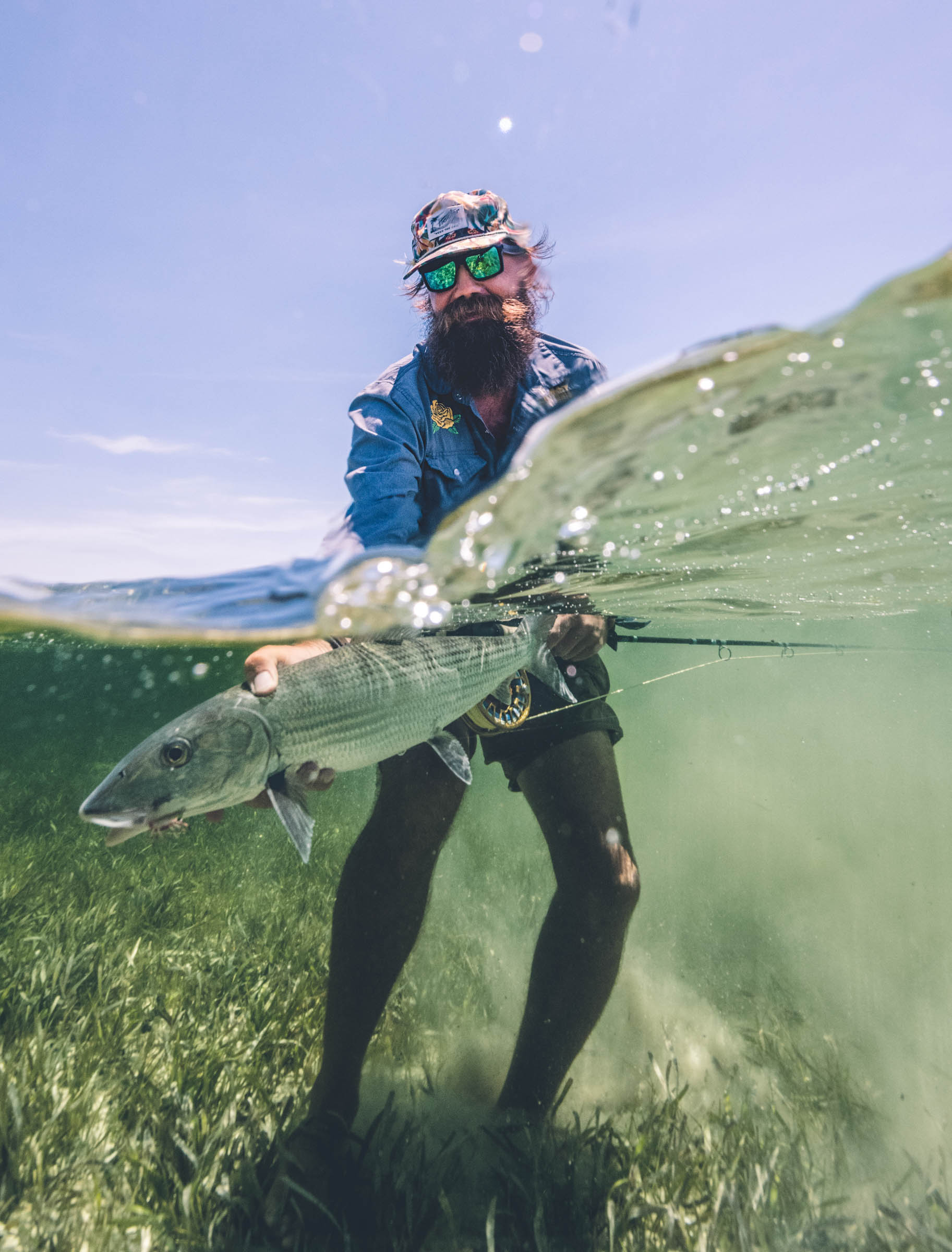The image depicts a fisherman standing in a shallow ocean reef, half-immersed in greenish, transparent water with bluish hues on the left side. It is a portrait-oriented color photograph showcasing partially underwater and above-water perspectives. The fisherman, a bearded and sun-tanned Caucasian man with a substantial mustache, is wearing reflective green sunglasses, a blue denim jacket, and a fisherman's hat. He is facing the viewer and looking slightly downward. In his hands, partially submerged, he holds a grey barracuda with a lure in its mouth, indicating he caught it using his fishing rod, which is visible in the background along with black tights he is wearing. The fish, appearing alive, is angled with its head towards the bottom left and its tail toward the fisherman. The water on the right side appears slightly blurred, possibly due to the fisherman treading and disturbing the ground surface. The sky above is blue, with grass-like structures visible at the bottom left of the image, emerging from the ocean floor covered in green coral. The style of the photograph is representational realism, capturing the dynamic interaction between the fisherman and his aquatic surroundings in a moment of underwater adventure.